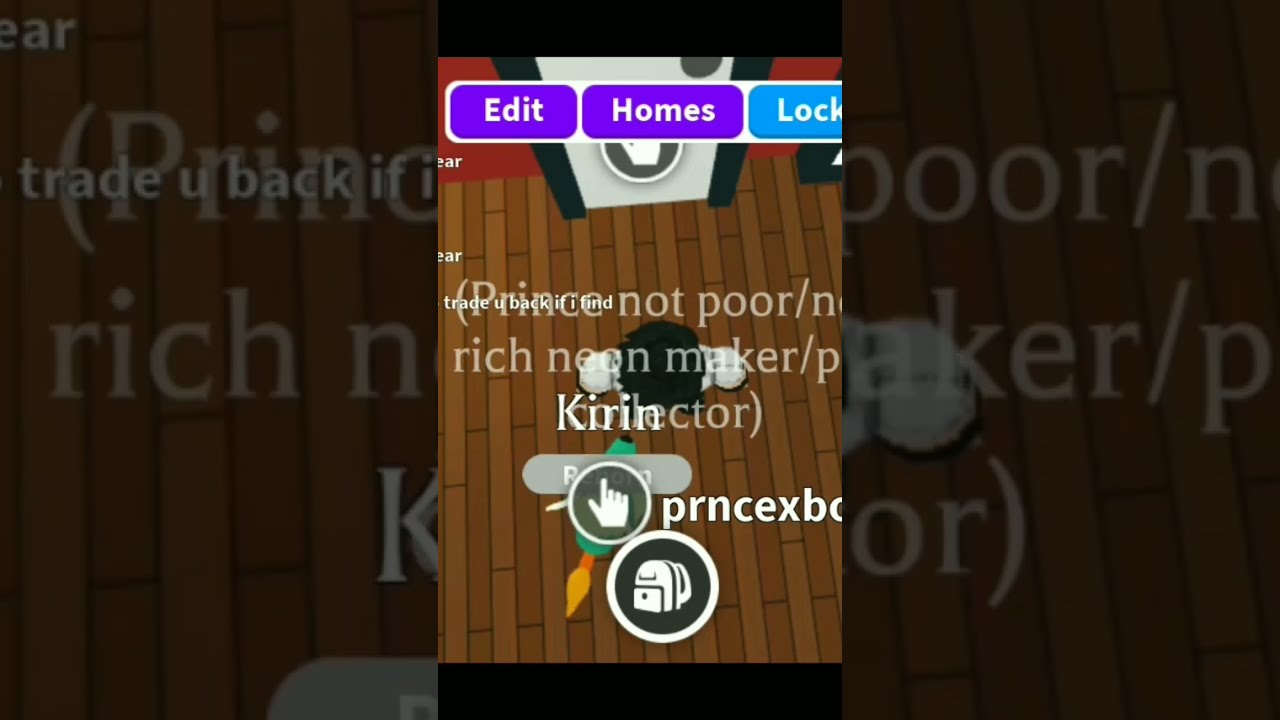The image is a detailed screenshot, possibly from a website or a mobile game, with a predominantly brown background. Centrally positioned, there are three prominent tabs at the top: the first two tabs are purple with white letters reading "Edit" and "Homes," while the third tab is turquoise with white letters reading "Lock." Below these tabs, text reads "Prince Not Poor, Rich Neon Maker, Curen, PRNCEXBC," overlapping with text behind it, creating a jumbled effect. The image also features a circle with a finger icon and, beneath that, a black circle depicting a white backpack in its center. This primary image is placed against a backdrop of an identical, but darker and filtered, version of the same slide, forming a composite visual layout. The background features a dark theme with text elements including "trade you back," "rich," further emphasizing the central content. Overall, the scene appears as a layered computer screenshot or screenshot of an advertisement with multiple text and button elements.